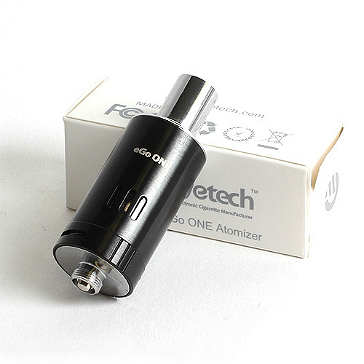The image, a color photograph in landscape orientation, prominently features a sleek cigarette atomizer resting diagonally on a white cardboard packaging box with gray text. The atomizer is a small, black cylindrical object with a shiny metallic screw attachment at the bottom and a silver cap at the top. The black body of the device displays the logo "EGO-1" in white text near the upper section. The light in the photograph is bright, highlighting the atomizer and casting a nearly blinding white glow across the scene. The packaging underneath, printed with the words "One Atomizer" and partially obscured lettering, reinforces the atomizer's presentation as a neatly designed product, emphasizing its functional and aesthetic features through detailed and high-realism product photography.